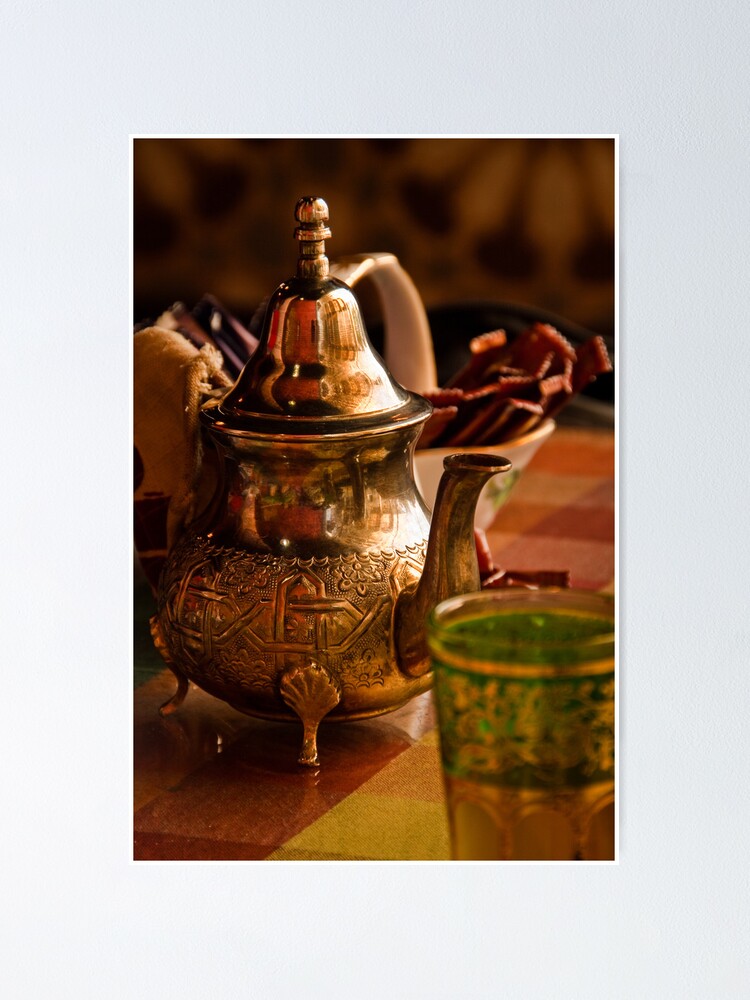The image captures a highly detailed and ornate teacup set, a central focus of the scene. The teacup, appearing to be very old and elegant, is predominantly made of a shiny, reflective brass or copper material that exhibits a golden-bronze hue. It features intricate etching on its bottom half and stands on four small, ornate legs. The top part of the teacup resembles a bell shape and is highly reflective, adding to its opulent appearance. The teacup also has a prominent, elegantly designed spout and a large handle. 

In the background, slightly out of focus, sits a white porcelain bowl containing what look like meat sticks or a similar type of food. The table on which the teacup rests is composed of red, yellow, and pink speckled squares arranged in a grid pattern, giving it a vibrant, mosaic-like look. Additionally, in the bottom right corner of the image, a blurry glass cup with a green and gold shading is partially visible. The entire image is bordered by a white frame, smoothly drawing the eye towards the central teacup, which remains the focal point of this elegant and formal table setting.